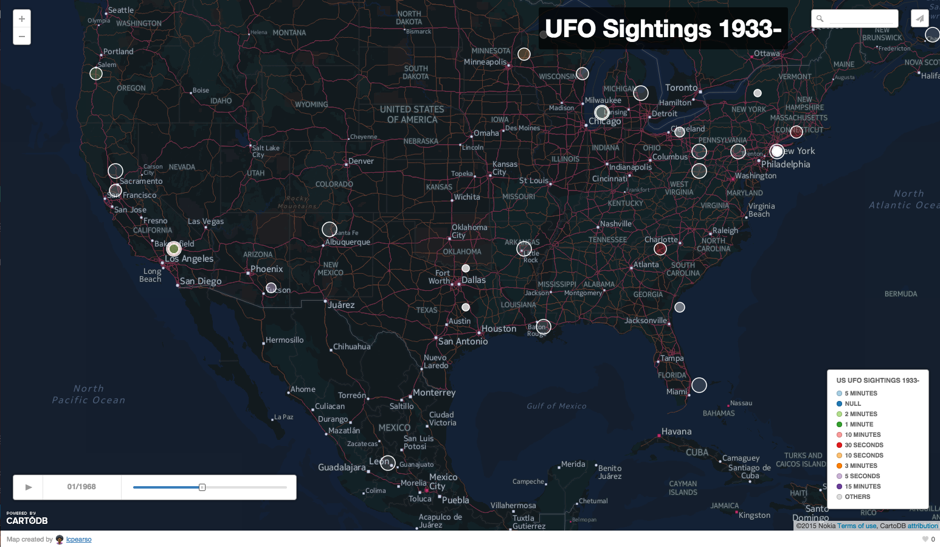This image is a dark-hued map of the United States, depicting UFO sightings from 1933 to the present. The map’s background, including the water bodies like the Atlantic Ocean, Pacific Ocean, and the Gulf of Mexico, is shaded in deep blue to nearly black tones. 

A key feature of the map is a timeline at the bottom with a play button, allowing users to view the chronological progression of UFO sightings. As the timeline progresses, markers representing UFO sightings appear throughout the map. 

In the bottom left corner, there is a legend explaining the markers, which are color-coded based on the duration of sightings, ranging from a few seconds to several minutes. However, many sightings are brief, often listed as only a few seconds or minutes, such as "3 minutes" or "30 seconds". 

The distribution of sightings is uneven, with fewer reports from the Midwest, while the Northeast shows a relatively higher frequency of events.